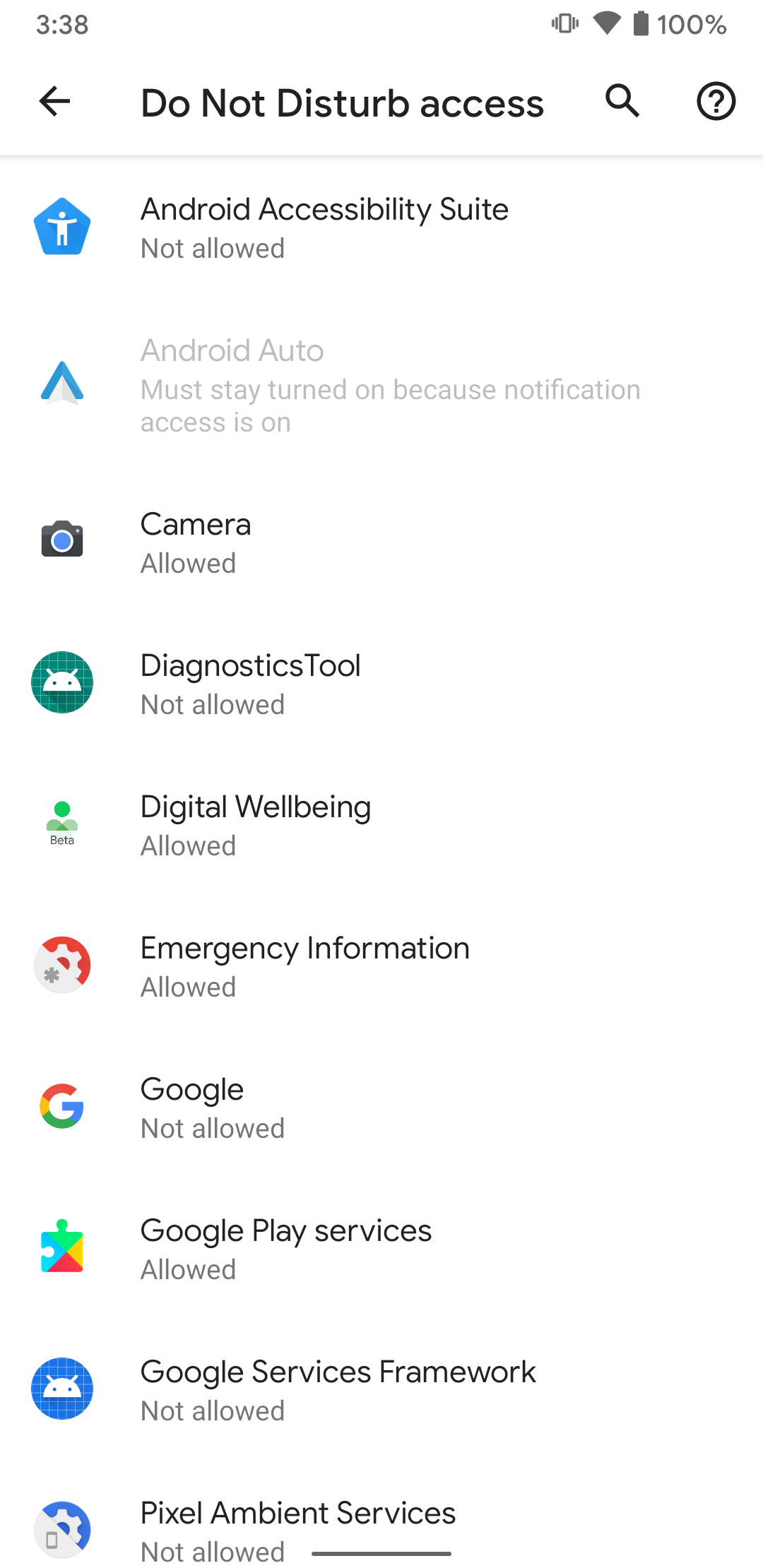This image is a detailed screenshot taken from an Android smartphone, specifically displaying the "Do Not Disturb Access" settings. The top left corner of the screen shows the time as 3:38 in light gray text. The status bar also indicates that the device has full Wi-Fi signal strength and a fully charged battery at 100%, denoted in light gray at the top right corner.

Directly beneath the status bar on the top left is a black left-pointing arrow for navigation back to the previous screen. To its right, in bold black text, it reads "Do Not Disturb access." Adjacent to this text are two icons: a search icon and a question mark icon, both also in black.

Further down, the screen enumerates the apps that have varying "Do Not Disturb" permissions. Each app's name appears in black text, accompanied by its status—either "allowed" or "not allowed"—written in light gray. The apps listed from top to bottom include:

1. **Android Accessibility Suite** – Not allowed (icon: A blue pentagon surrounding a figure with outstretched arms)
2. **Android Auto** – Must stay turned on because notification access is on (icon: A blue upward arrow)
3. **Camera** – Allowed (icon: A camera)
4. **Diagnostics Tool** – Not allowed (icon: A green circle containing the white head of a creature)
5. **Digital Well-being** – Allowed (icon: A green figure with a halo)
6. **Emergency information** – Allowed (icon: A red settings cog)
7. **Google** – Not allowed (icon: The multi-colored 'G' logo)
8. **Google Play Services** – Allowed (icon: Not explicitly mentioned)
9. **Google Services Framework** – Not allowed (icon: Not explicitly mentioned)
10. **Pixel Ambient Services** – Not allowed (icon: Not explicitly mentioned)

The background of this settings screen is white, providing a clean visual contrast to the black text and various icons associated with each application.